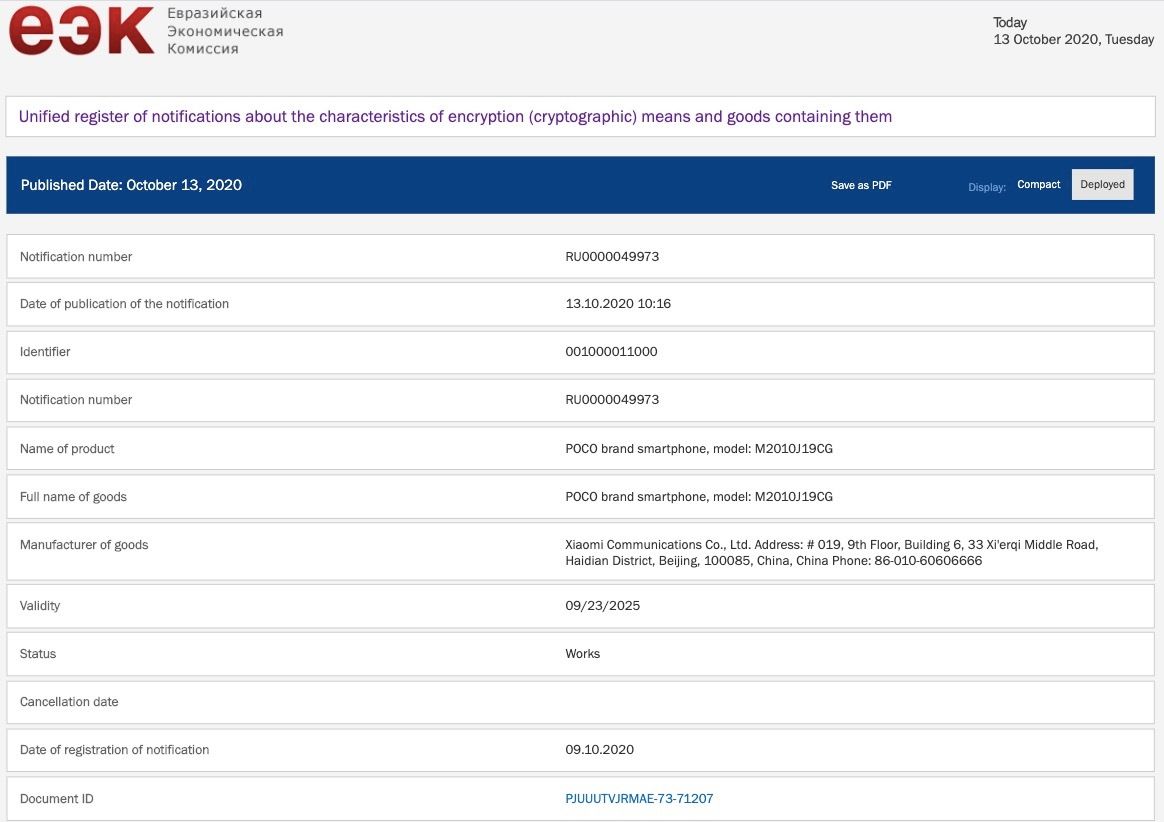This is a detailed description of an image of a website, predominantly in Russian, with English elements. At the top of the site, there's text that appears to be a mix of Russian and English, beginning with an English "E," followed by a backwards capital "E" with curves, a capital "K," a lowercase "e," and some Russian text that is not readable. The site displays the following English text: "Today, October 13, 2020, Tuesday, unified register of notifications about the characteristics of encryption, cryptographic means and goods containing them." Below this, there is a blue header bar that spans the width of the screen.

This header includes information: "Published date: October 13, 2020," options to "Save as PDF," and a display mode toggle between "Compact" and "Deployed." Below the header, there is notification number "RU0000049973," displayed in thin, outlined rectangular fields running the full width of the screenshot. 

The image lists the following details:
- Date of publication of the notification: 13.10.2020 at 10:16
- Identifier: a string of zeros and ones
- Notification number: RU0000049973 (repeated from above)
- Name of product: Poco brand smartphone, model M2010J19CJ
- Full name of goods: Same as above
- Manufacturer of goods: Xiaomi Communications Company, with their address included (not specified here)
- Validity: Until 23-09-2025
- Status: Works
- Cancellation date: Blank
- Date of registration of notification: 10-09-2020
- Document ID: An alphanumeric string in large blue text

All this information is organized neatly within the webpage, with each detail aligned within the described fields.